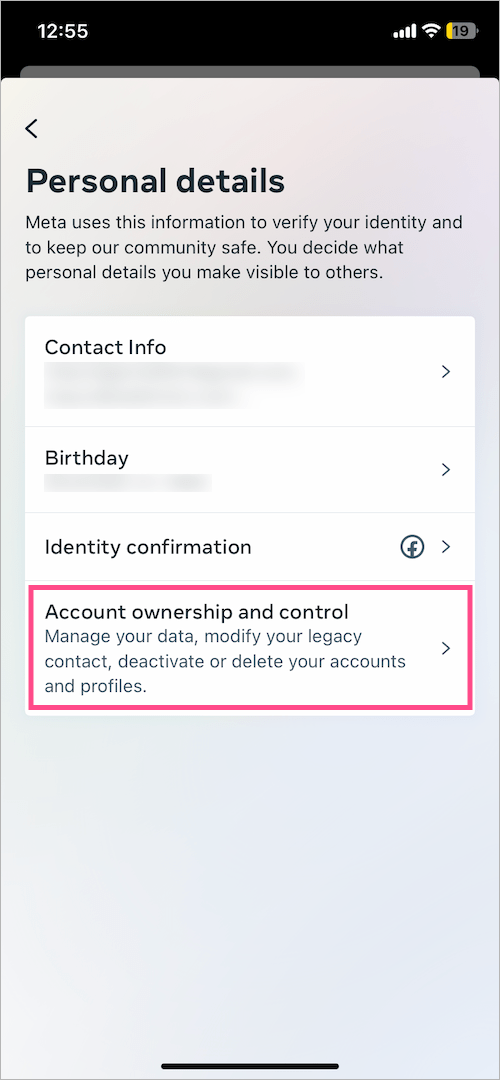The image is a screenshot from a cell phone depicting a user interface. At the top of the screen, there is a black banner displaying the time "12:55" in white text. To the right of the time, icons for cell signal strength, Wi-Fi connectivity, and battery status are shown; the battery icon contains a yellow segment indicating it is at 19% charge.

Beneath the banner, the background is gray with a left-pointing arrow, followed by the title "Personal Details" in capitalized black text. Below this heading is a description in smaller text: "Meta uses this information to verify your identity and to keep our community safe. You decide what personal details to make visible to others."

Further down, there is a blurred section labeled "Contact Info" with a right-pointing arrow next to it, indicating more details can be accessed. Below that, another blurred section labeled "Birthday" also has a right-pointing arrow.

The section for "Identity Confirmation" features a circle with an "F" inside it and another right-pointing arrow. Highlighted within a pink rectangle is the heading "Account Ownership and Control," which includes options to manage data, modify legacy contacts, deactivate, or delete accounts and profiles, with yet another right-pointing arrow adjacent to it.

Finally, a black line runs along the bottom edge of the screen.